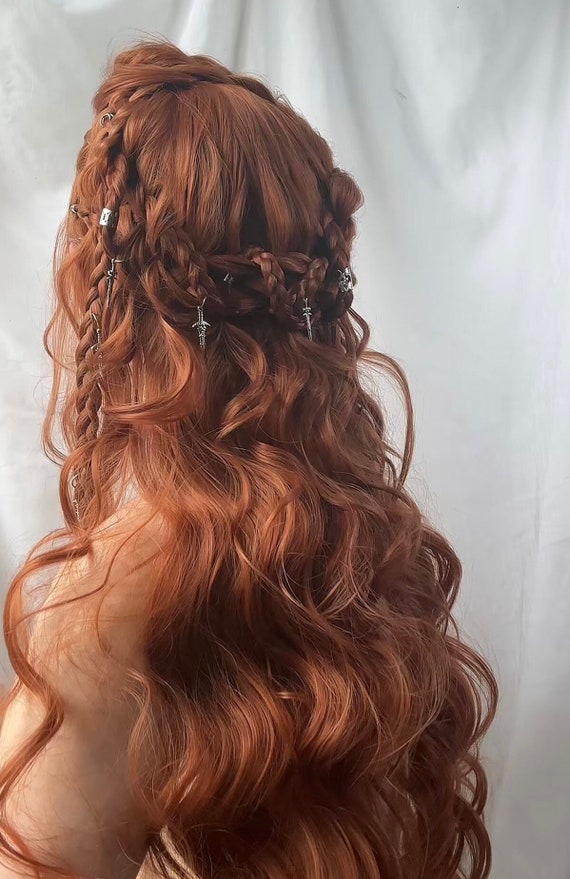The image captures the back of a woman with striking, long dark red hair, styled impeccably for what suggests a special event, possibly a wedding, as she might be a bride or participant. The main focus is on her intricate hairstyle: her hair cascades down her back in loose waves, complemented by a sophisticated braid that forms a halo around the upper part of her head. This primary braid, along with an additional solo braid running vertically down her left side, is adorned with medieval-inspired silver charms, including crosses and daggers, intricately woven through at two-inch intervals. She stands before a white, textured background that resembles a curtain, gently ruffled towards the top. Her head is turned to the left, facing away from the camera, and only her bare left arm is visible, suggesting she might be wearing a sleeveless garment or one that ties around the neck. The detailed elegance and placement of the braids and charms underscore the meticulous effort put into her hairstyle.